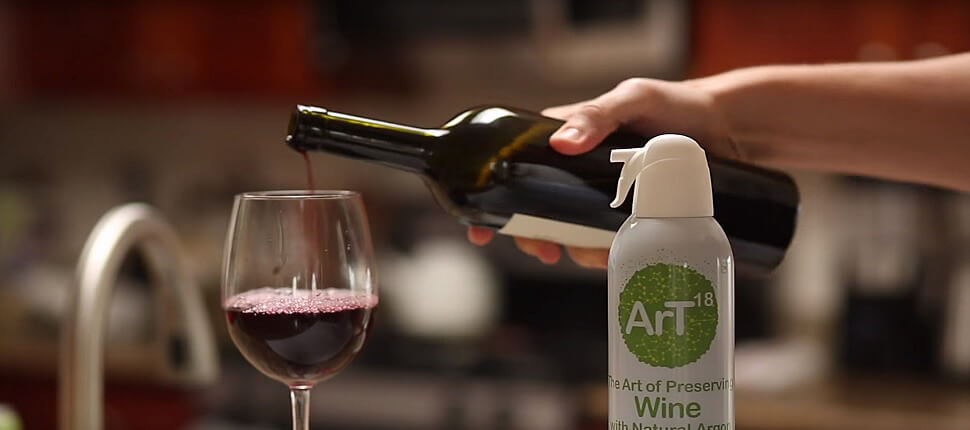This colored photograph, set in a kitchen, captures a white hand pouring red wine from a bottle into a quarter-full white wine glass. Prominently displayed in the foreground is a spray can labeled "Art 18, the art of preserving wine with natural aromas," featuring a white background with green lettering and a green circle. The bottle, can, and glass are sharply in focus, while the background, which includes a kitchen faucet, stove, microwave, and dark mahogany cabinets, is blurred. The image suggests the use of the Art 18 product to help preserve wine at home, ideal for those who do not wish to finish their entire bottle in one sitting.